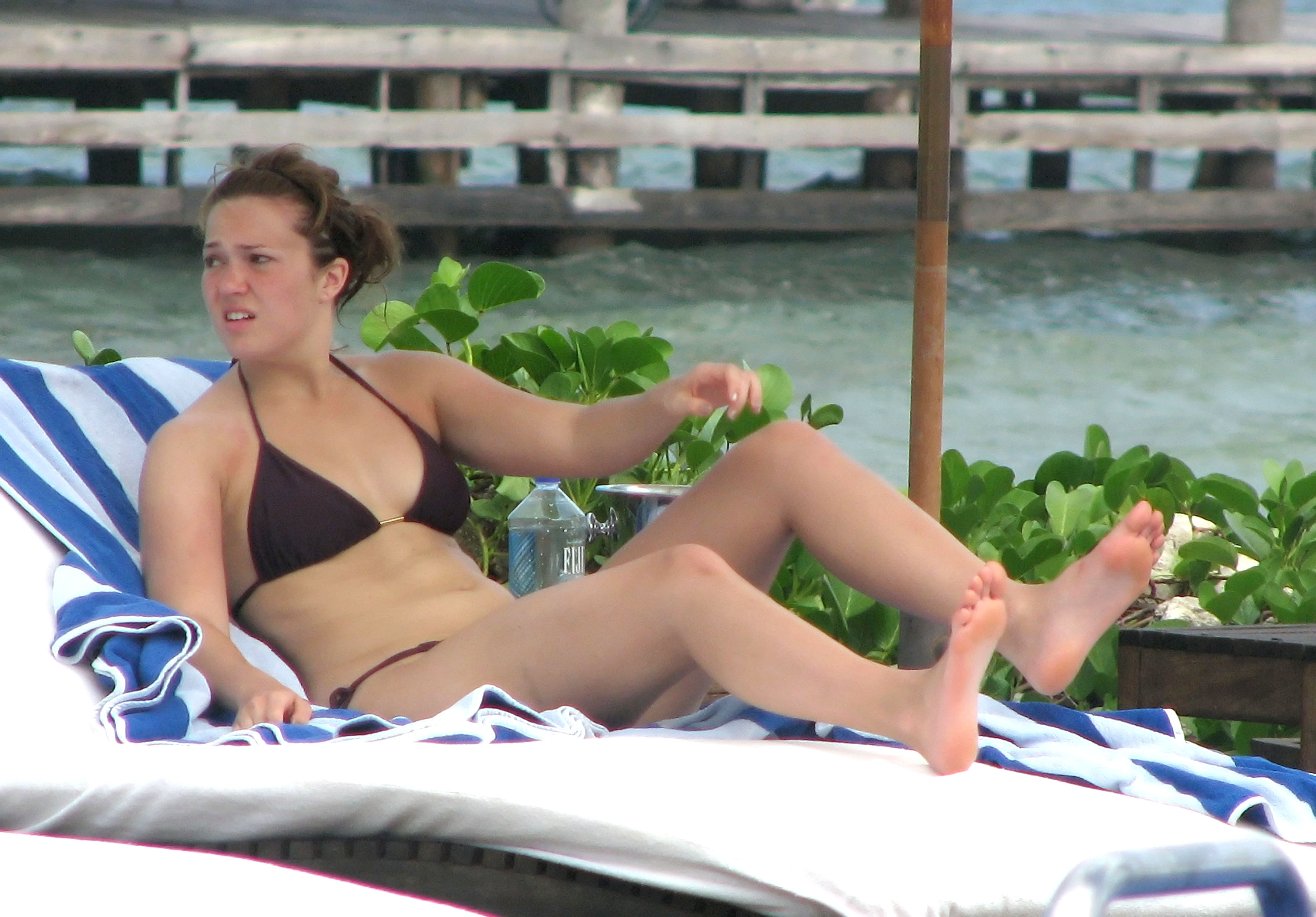This horizontal rectangular photograph captures a young woman in her 20s sunbathing beside a greenish-brown lake. She is reclining on a white chaise lounge, which is covered with a blue and white striped towel. The woman's hair is long but pulled up in a messy bun, and she wears a skimpy black triangle halter bikini. She is looking over her right shoulder with a slightly anxious or searching expression, her mouth slightly open, and her left hand held slightly in the air. Her feet are slightly raised, adding to her relaxed yet alert pose. Beside her on the chair is another towel and a plastic Fiji water bottle. 

In the background, there's a lush display of greenery and planters with green leaves next to her. The scene extends further to reveal a pier or dock made of wood at the top of the image. To the woman's left, there is a pole near her shin, likely supporting an umbrella. This serene lakeside setting is complemented by buildings visible beyond the lake, suggesting a blend of natural and built environments.